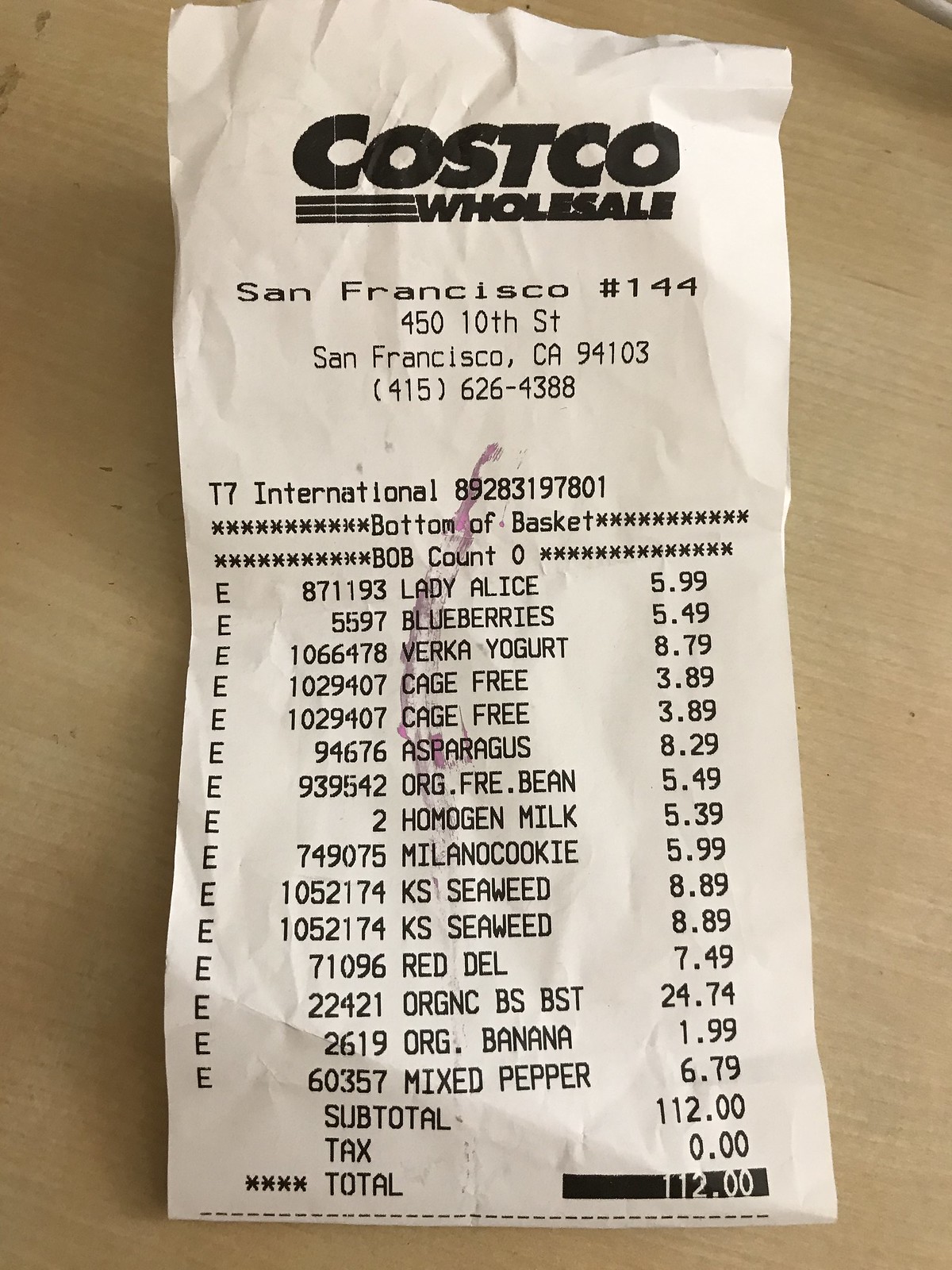This image captures a detailed Costco receipt, neatly placed on a beige countertop. The white receipt features black text and a distinct small purple line running through it. At the top, it clearly displays "Costco Wholesale" followed by the location in San Francisco, California, alongside the store's address. Each purchased item is meticulously itemized, including apples, blueberries, yogurt, eggs, asparagus, beans, milk, cookies, seaweed, more apples, an unspecified item, bananas, and mixed peppers. The subtotal reads $112, with no additional tax, resulting in a grand total of $112. The image excludes any people and contains no text beyond the details printed on the receipt, ensuring the focus remains solely on the documented purchases.